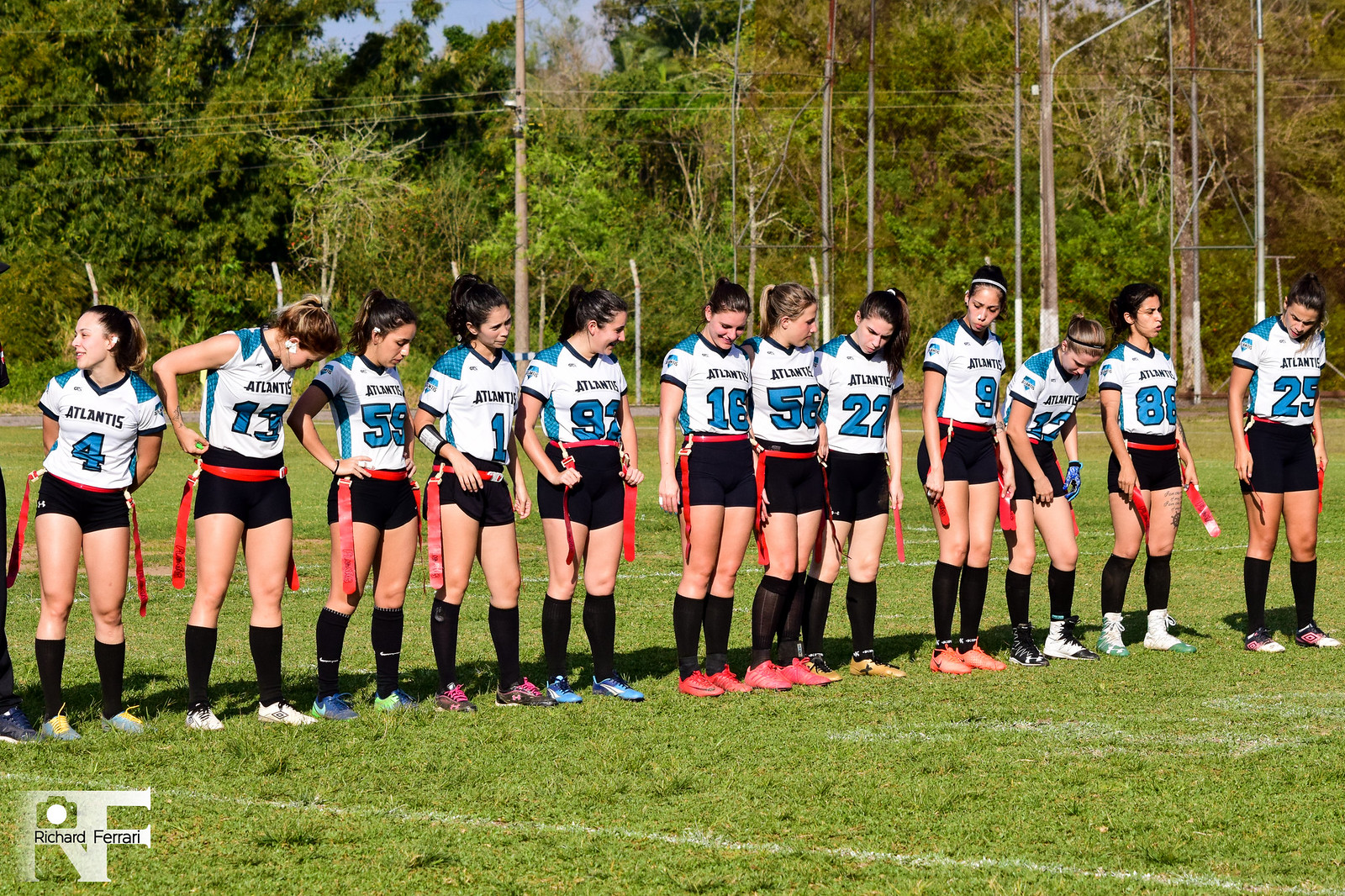The photograph features a lineup of women athletes in an outdoor flag football setting. They are positioned in a straight row on a grassy football field under daylight, with sunlight illuminating both the players and the lush green surroundings. The blue sky is partially visible in the background, along with trees, some of which have bare branches. Each athlete wears a white short-sleeved jersey with blue trim and the name "Atlantis" emblazoned on the front, accompanied by their distinctive team numbers in blue with black borders. Their uniform includes black shorts, long black socks, and red flags secured around their waist. The jersey numbers range from 1 to 97, including 4, 13, 55, 16, 58, 27, 9, 12, 88, and 25. The bottom left corner of the photograph features a logo with the letters "R&F" and a camera design, accompanied by the name "Richard Ferrari."